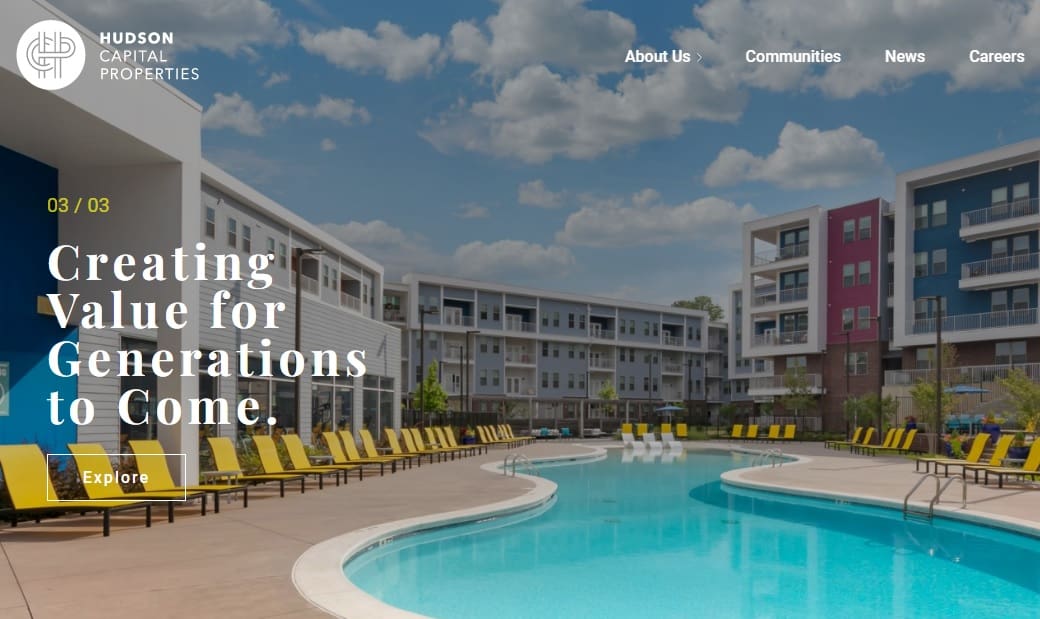This vibrant image serves as the homepage of a Hudson Capital Properties website. The layout is approximately 50% wider than it is tall, providing a panoramic view of a luxurious pool area. The pool itself is uniquely designed with three tiers, reminiscent of a multi-layered hourglass. The tiers become progressively narrower as they ascend, creating an elegant and sophisticated visual effect.

Surrounding the pool are a collection of about 30 yellow lounge chairs, meticulously arranged in a symmetrical pattern. Approximately 15 chairs line the left side, five are positioned at the far end, and another 10 occupy the right side, all perfectly poised for guests to relax and enjoy the serene environment.

In the background, a series of vibrant buildings add to the dynamic setting. The structures vary in color, featuring bold blue, striking red, sleek gray, and a subtle off-white, giving the scene a diverse yet harmonious appearance. These buildings could be hotel rooms, condos, or even timeshares, contributing to the luxurious atmosphere.

Above, the sky is a picturesque blend of blue with scattered clouds, suggesting a pleasant daytime setting. 

Overlaying this picturesque scene, the upper left corner of the image features the logo and name of "Hudson Capital Properties," while the upper right corner displays navigation controls for easy access to various sections of the website such as "About Us," "Communities," "News," and "Careers." Centrally placed on the left side is the company's inspiring slogan, "Creating value for generations to come," encapsulating their long-term vision and commitment.

This detailed visual presentation effectively combines elements of luxury, comfort, and corporate professionalism, making it an engaging and inviting homepage.